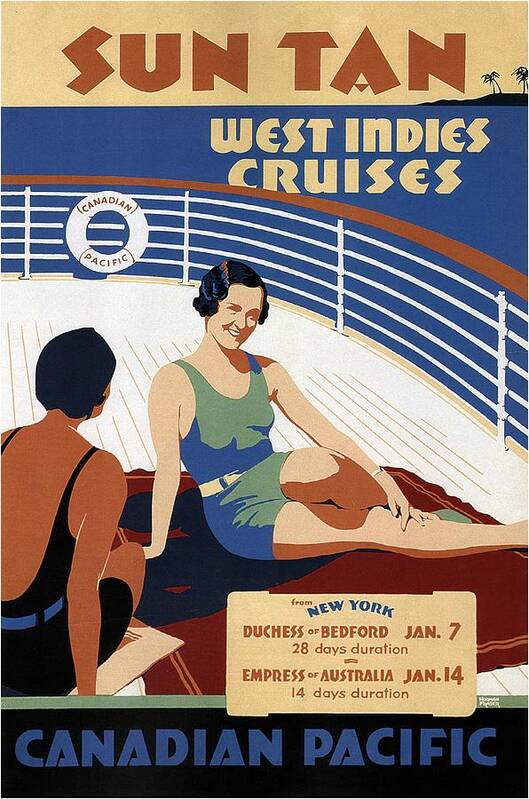This visually captivating tourism poster, designed with an homage to the vintage aesthetic of the 1930s through 1950s, radiates an Art Deco charm. It presents a scene set on the deck of a cruise ship, with the muted tones of blues and yellows evoking a nostalgic feel. At the top of the poster, "Sun Tan" is inscribed in a maroon or burnt orange color, followed by "West Indies Cruises" in beige, complemented with the depiction of serene palm trees against a blue backdrop symbolizing the ocean.

The deck itself is a pristine white, bordered by a railing and featuring a life preserver emblazoned with "Canadian Pacific." Two women, one with a light complexion in a green swimsuit and another darker-skinned woman in a black swimsuit, are leisurely strewn across the deck. They are wearing modest one-piece swimsuits evocative of an earlier era, enhanced by the retro touches akin to shorts. One lounges on a red towel while the other reclines on a tan one; one of the women faces the camera with a smile, while the other is turned away, adding a natural, candid feel to the scene.

At the bottom, set against a black background with blue fonts, the text highlights the travel details: voyages from New York via the Duchess of Bedford, starting January 7th for a 28-day duration, and the Empress of Australia departing January 14th for a 14-day journey. The overall muted color palette and intricate period details make this modern recreation a fitting tribute to classic travel advertising.